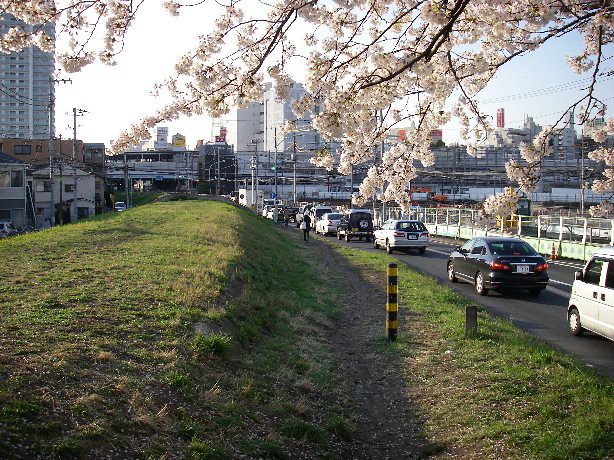This vivid outdoor scene, captured on a sunny day, appears to be near a downtown area. The foreground features a grassy hill that slopes down toward the center of the image, transitioning into a bustling road on the right side. The road is lined with a series of cars caught in what seems like traffic, and a man can be seen walking along the road's edge, though it's difficult to discern whether he is on foot or biking.

Dominating the scene is a beautiful tree adorned with white flowers, positioned prominently from the top right corner and spreading its branches gracefully. The middle ground is populated with various buildings, ranging from tall city structures to smaller residential houses, suggesting a cityscape. Notable in the mix is a very tall, tower-like building on the left side, while power lines stretch across the scene, adding to the urban ambiance.

A white fence follows the road on the right, juxtaposed with a short, black-and-yellow striped pole that stands about as tall as the cars. The colors in the image are diverse, spanning green, brown, yellow, black, white, gray, red, tan, and pink, contributing to a lush, vibrant atmosphere. The sky above is crystal clear, free from clouds, emphasizing the brightness of the setting.